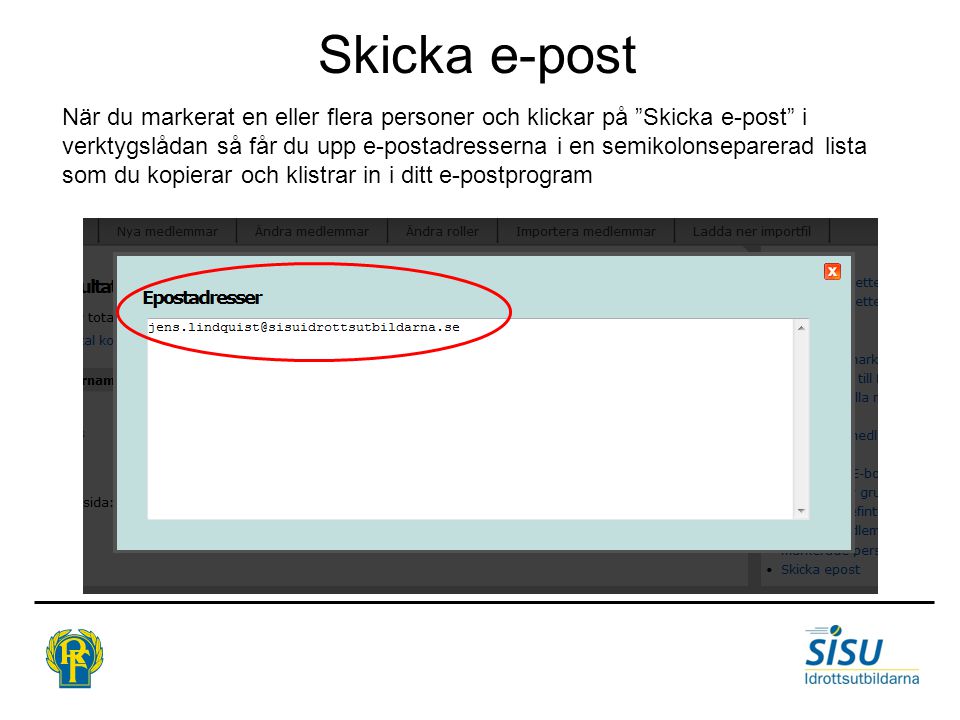The image is a screenshot of a computer application, likely a PowerPoint presentation or a similar app, with text predominantly in an unfamiliar foreign language. The title at the top reads "Skicka e-post," which appears to be Swedish. Beneath the title is a small paragraph of black text describing some aspects of the application. A key feature in the middle of the screenshot is a blue rectangular window with "e-postadresser" written above a text box, which contains the email address "gens.linquist@sisuidrottsutbildarna.se," circled in red. In the upper right corner of this window, there is a red square icon with a white X. The bottom right corner of the image displays the blue and white logo "SISU, Idrottsutbildarna," and the bottom left corner features another logo labeled "RF" in blue and yellow.